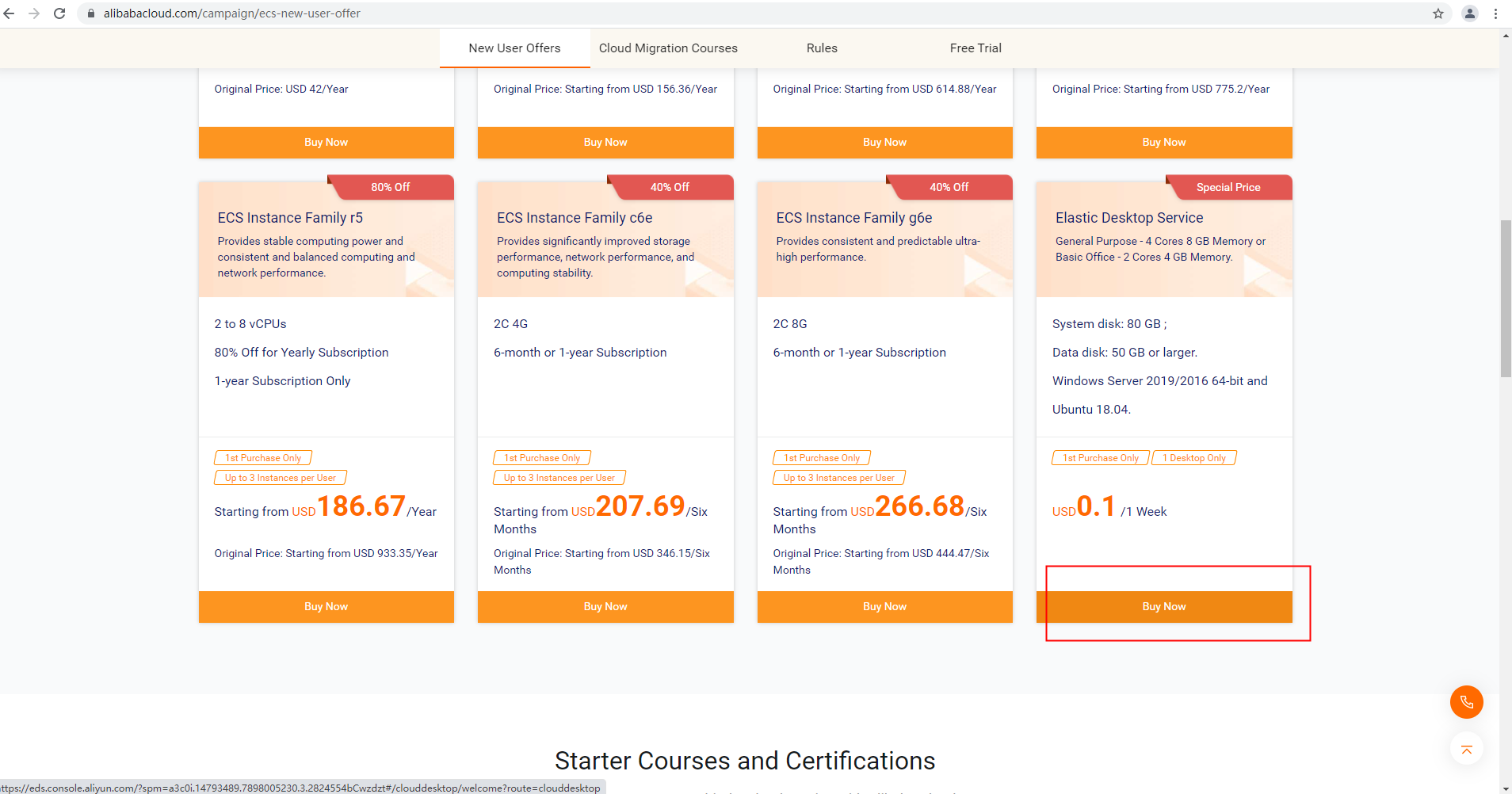This screenshot features a detailed view of a desktop browser window accessing a promotional page on Alibaba Cloud. At the top, the address bar is visible, in shades of white and light gray, with navigation elements including a gray left arrow, a lighter gray right arrow, a gray refresh button, and a lock icon next to the URL: alibabacloud.com/campaign/rec-new-user-offer. Below, a light grayish-peach colored navigation bar showcases tabs labeled "New User Offers" (currently selected), "Cloud Migration Courses," "Rules," and "Free Trial."

The main content area displays a grid of eight promotional categories arranged in four columns with two cards per column. The top row of cards is partially cut off, while the bottom row is fully visible. Each card features an orange "Buy Now" button at the bottom, with product details presented above.

On the right-hand side of each card, red banners highlight discounts stating "80% off," "40% off," "40% off," and "Special Price." Within the cards, peach-colored headers designate product types such as "ECS instance family R5," "C6E," "G6E," and "Elastic Desktop Service."

A white text box in each card provides additional course details. Below this, two orange-bordered boxes contain further information in orange lettering. Price details are listed across the bottom of the cards as follows: $186.67, $207.69, $266.68, and a unique price of USD 0.1. Each card ends with an orange "Buy Now" button, with the last one on the bottom right partially obscured by a red-outlined clear box stating "Starter courses and certifications" in black.

At the very bottom right, an orange bubble featuring a white phone icon is displayed, along with another white bubble containing an additional icon, indicating customer support options.